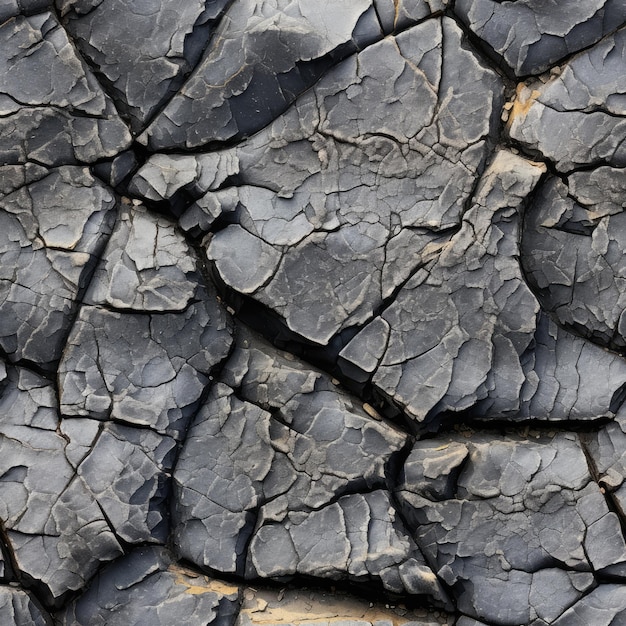This close-up image displays a highly detailed, magnified view of a gray stone wall with numerous cracks and fissures, creating a scaly and fragmented appearance. The stone surfaces are varied in shape, uniformly light gray, with some sections reflecting light, giving them a shiny, almost metallic or whitish sheen. The intricate network of ridges and lines resembles dried, cracked earth or the desiccated skin of an animal, adding an enigmatic, dramatic quality to the texture. The close-up composition limits the view to the immediate surface, heightening curiosity about the larger context of this cracked, scaly stone expanse.